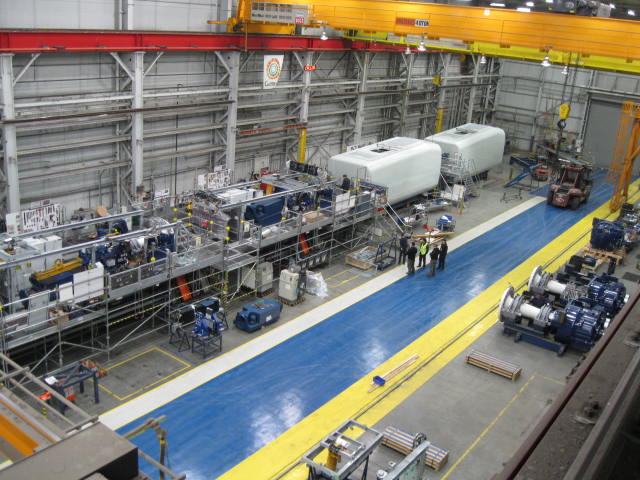The photograph captures a detailed view of a large factory interior with tall ceilings, taken from an elevated vantage point looking down. The building has a utilitarian, rectangular structure with aluminum walls lined with extensive scaffolding. Prominently featured are two beams: a red horizontal beam intersecting with a large yellow one, suggesting a crane mechanism. An orange crane track runs across the top right of the image, with visible red tracks indicating its movement path. The factory floor is marked with a blue stripe running diagonally from the lower left to the upper right, flanked by a yellow stripe below and a white stripe above it. On the right side of the floor, several large engines or rocket-like machinery are situated, with a forklift visible in the background. In the center of the image, four people are surrounded by various equipment and machinery, hinting at ongoing construction or production activities.